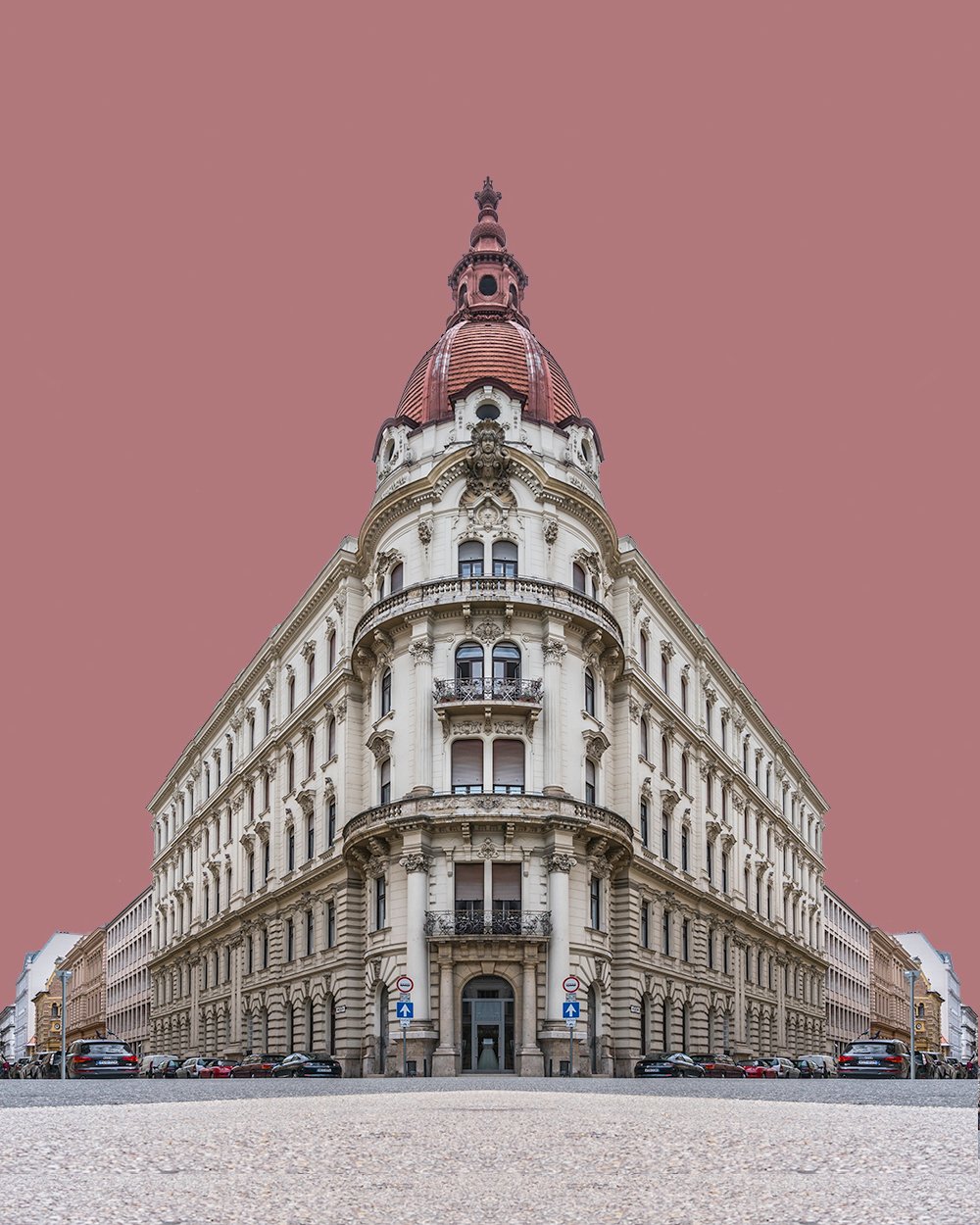The image showcases a striking, old triangular-shaped building prominently located at the intersection of two busy streets, underscored by its distinct architectural features. The building, possibly a grand hotel, department store, or even a palace-like structure, stands five to six levels high, crowned with a large dome and spire at the acute-angled tip of the triangle. Windows line the entirety of the building's facade, and a set of ornate artwork is displayed just below the dome. At street level, a prominent doorway nestled under an archway marks the entrance, flanked by pedestrian crosswalk signs.

Surrounding the building are numerous cars, parallel-parked along both intersecting streets, which feature pavement leading up to and around the structure. The ground is gray, and arrow signs direct traffic straight ahead, with parking meters visible on the sidewalks. The sky above is a solid reddish-brown, possibly due to a filter, giving the scene an ominous feel. Despite the sky's dramatic hue, reflections in the car windows suggest it is daytime. The entire setting is vividly captured in an outdoor environment, free from any text or other distractions.